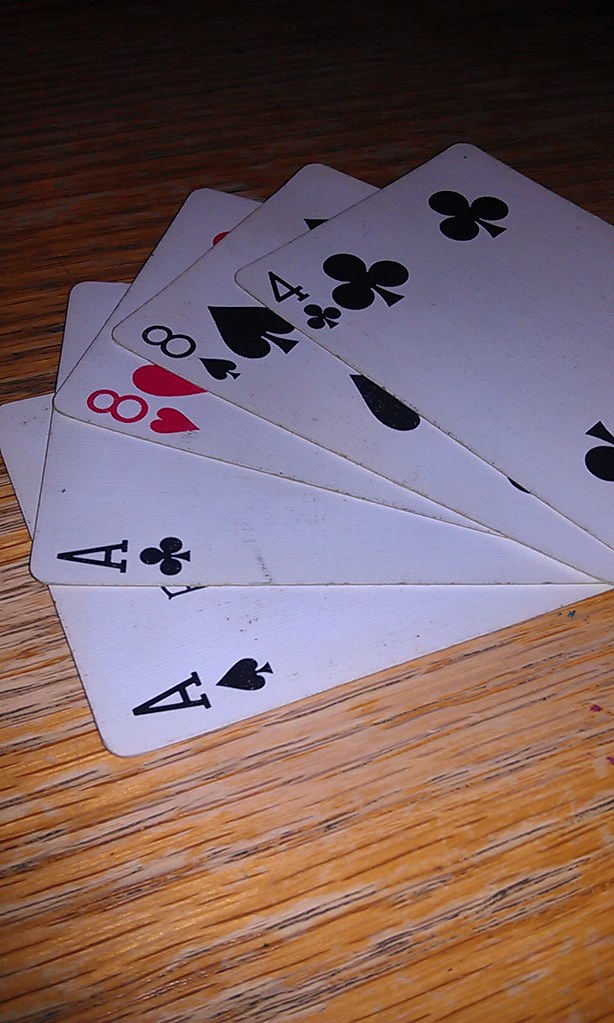On a distressed wooden table featuring a mix of reddish, light tan, and blackish wood grains, five well-worn playing cards are splayed out as if laid down after a poker game. The cards held in the image show a hand with two pairs: the Ace of Spades, Ace of Clubs, Eight of Hearts, Eight of Spades, and a Four of Clubs. The edges of the cards appear frayed, indicating their age and frequent use. The photograph was taken with a flash, illuminating the lower half of the image and gradually darkening toward the upper half. The table also bears subtle evidence of past markings or specks, adding to its rustic character. There is no text present in the image.